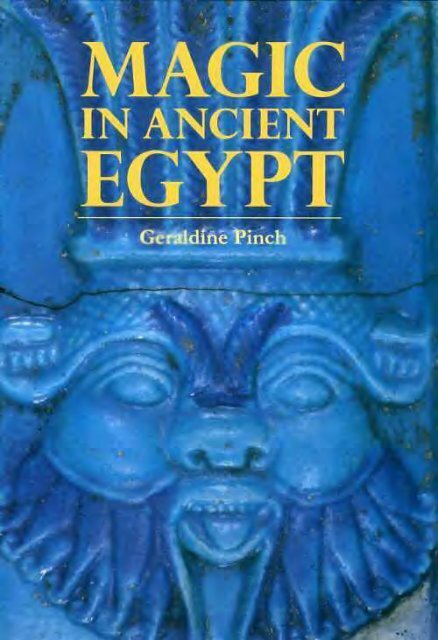The front cover of the book "Magic in Ancient Egypt" by Geraldine Pinch is predominantly blue, showcasing a striking image of what appears to be an ancient Egyptian mask or statue. The cover is detailed with varying shades of blue, giving depth to the carving's features. The title of the book is prominently displayed at the top in gold text, followed by a line, and beneath it, the author’s name, also in gold. 

The mask itself, occupying the lower half of the cover, depicts a face that doesn't look entirely human. It has an open mouth, a pronounced beard, and a broad nose. The head is crowned with what seems to be a headdress that features elements resembling feathers or horns emerging from the center. The details of the face are highlighted through the blue hues, while the overall composition gives a mystical and ancient feel. The mask appears regal, possibly that of a king or emperor, adding to the book's theme of ancient Egyptian magic.